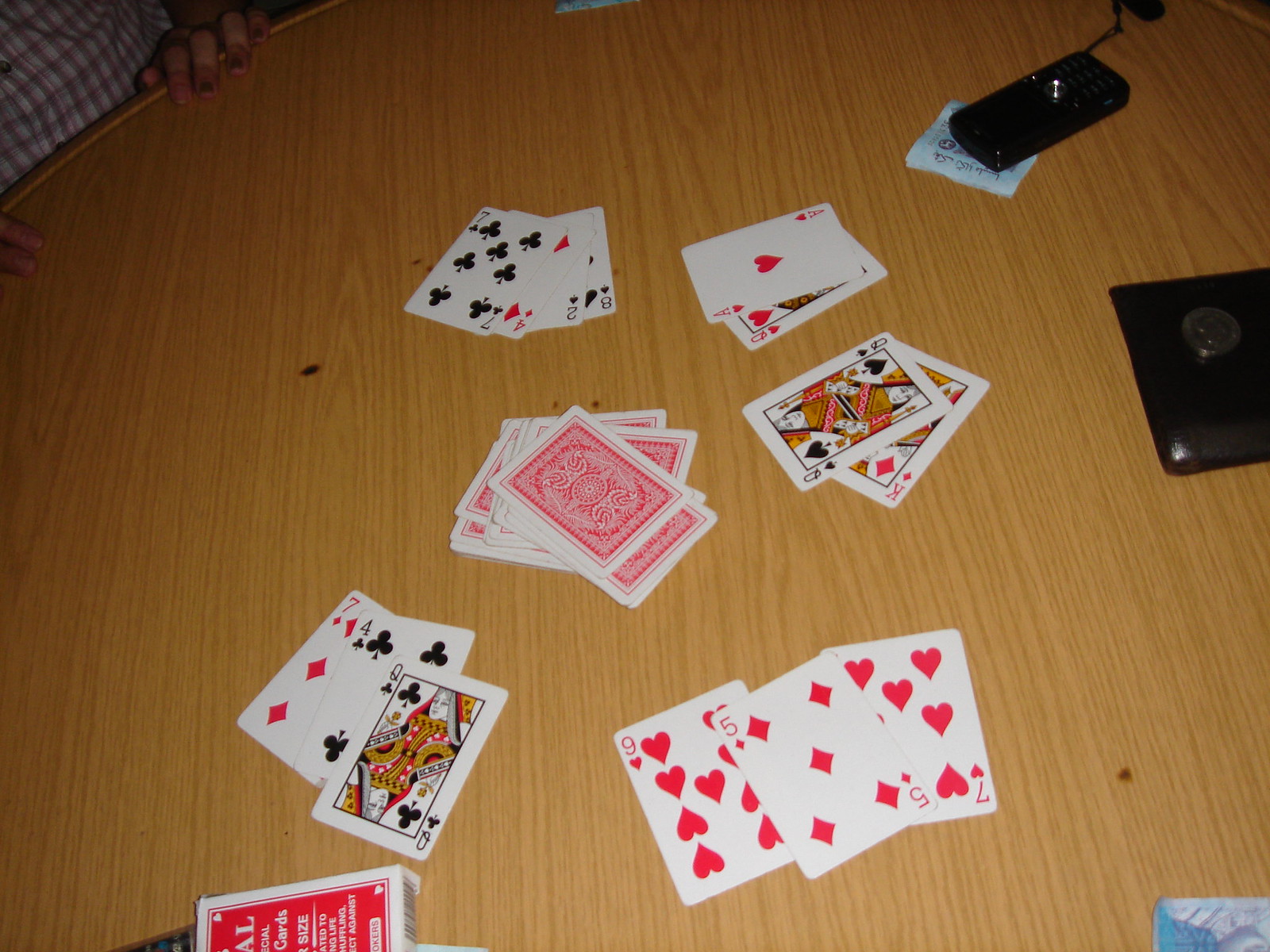The image showcases the interior of a bedroom with a scene centered around a wooden table of light brown color, featuring distinctive vertical lines. At the top left corner, a person’s hands are visible, grasping the table. The person appears to be wearing a checkered shirt with a white background and red stripes. Their fingernails are notably dirty; the left hand's three middle fingers have a black coloration, possibly from nail polish.

Prominently displayed in the middle of the image is the wooden table surrounded by various objects. Toward the top right, a black cell phone with a circular silver accent near the bottom stretches diagonally toward the bottom left. Slightly down and to the right sits an indeterminate object, either a square coaster or a leathery-textured wallet.

Scattered across the table, a variety of playing cards are seen in play. Notably, there are an 8, a 2, a 4, and a 7 in the middle-top left, an Ace and a Queen in the middle-top right, followed by another Queen and a King to the right. At the bottom left, there is a 7, 4, and a Queen, while the bottom right holds a 9, 5, and another 7. The scene suggests an ongoing card game amidst a casual setting.